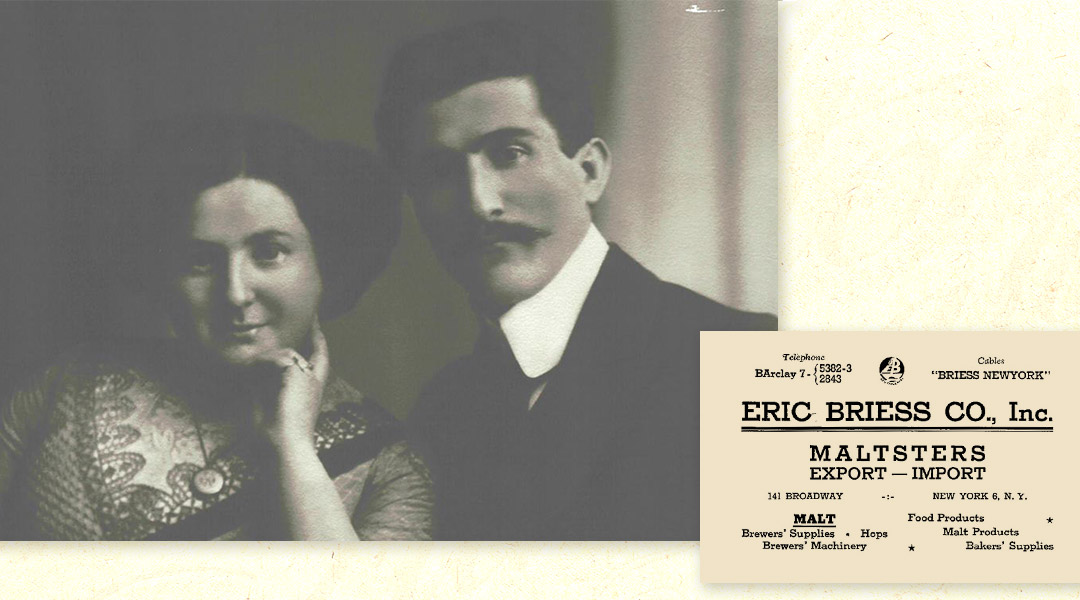A vintage black-and-white photograph captures a couple from their lower chest up, exuding an old-time charm. The man, dressed in a black suit jacket with a white collar, has dark hair and sports a thick mustache, reminiscent of historical figures like Nikola Tesla. Beside him, leaning in slightly, is a woman with dark hair that’s elegantly pulled up, wearing a detailed dress with a lace or crocheted neckline. She has a circular locket-type necklace and rests her left hand gently on her chin, adding a touch of grace with her subtle smile. This photograph, likely part of an advertisement, features textual information on the lower right corner: "Eric Bries Co., Inc. Maltsters Export-Import, 141 Broadway, New York." The text outlines an array of products offered by the company, including malt brewer's supplies, brewer's machinery, hops, food products, malt products, and baker's supplies, along with contact details such as a telephone number and cable address. The woman and the man, both slightly off-camera, give the image a timeless, classic essence while also serving a commercial purpose.